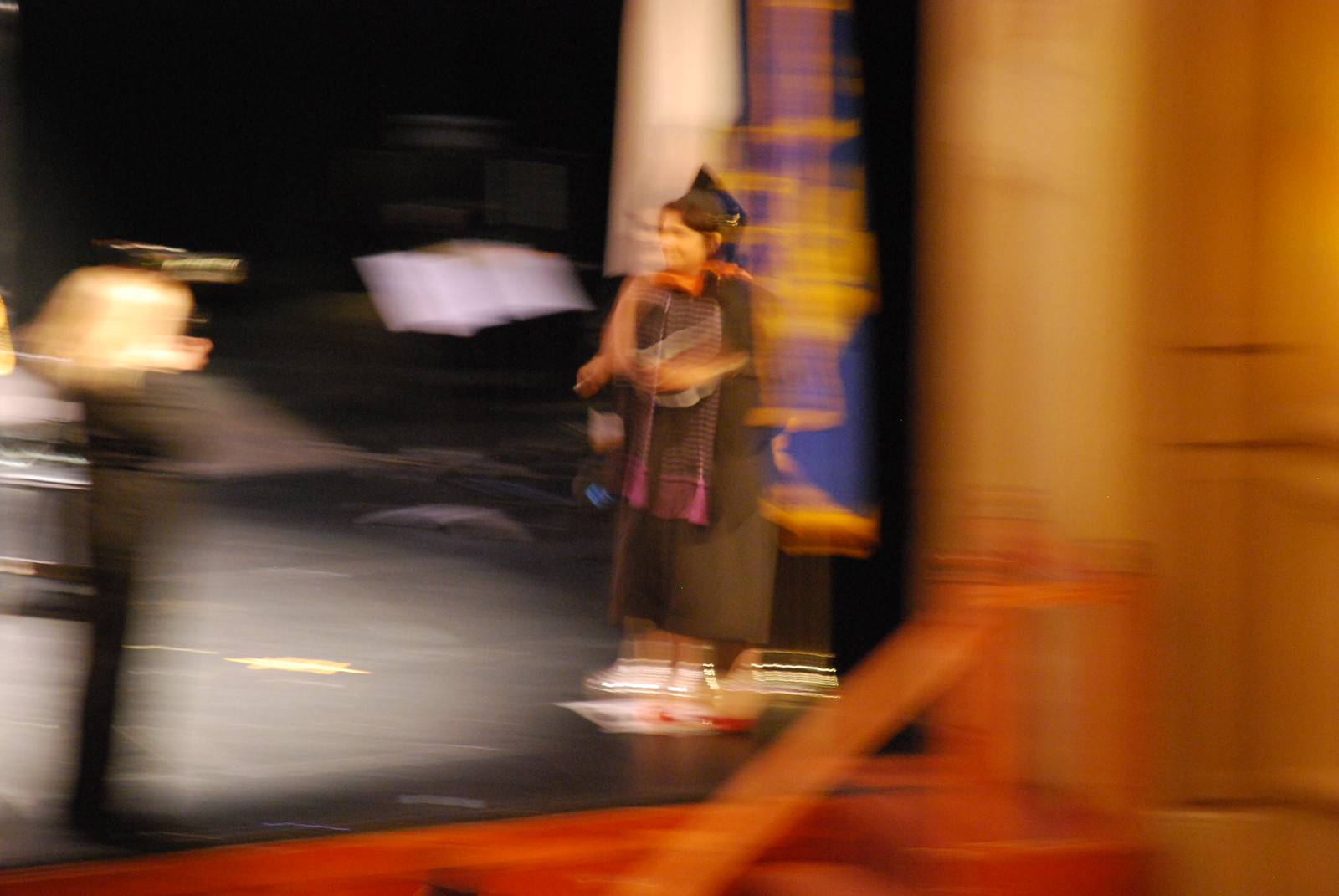A photograph captures the lively atmosphere of a graduation ceremony. On the right side of the image, a heavily blurred brown wall serves as a background, adding a touch of depth. The left side of the image is dominated by another indistinct black area, possibly another person blurred out by motion. The far left features a student with floating blonde hair, clad in a black gown and moving so quickly that their gown appears to be trailing behind. Next to this individual, another young woman stands out in sharp contrast. She is adorned in the traditional black graduation robe and cap, confidently carrying a blue flag embellished with gold details. Her determined stride takes her towards the left of the stage, where she is seemingly approaching the blonde-haired graduate. The beautifully chaotic composition of blurs and focused details perfectly encapsulates the excitement and fervor of graduation day.